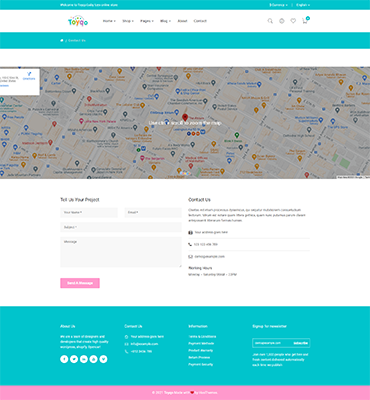The webpage appears to be for a company likely named "Toy Co." The header features a logo with text too small to clearly discern but seems to begin with "Toy." To the right of the logo, there are six tabs for site navigation, followed by four icon links. Below the header, there's an interactive map displaying various store locations for Toy Co. At the bottom of the page, there are several entry fields, though the purpose is unclear due to small text. To the right of these fields, a block of text is present, content of which is also unreadable. A green section follows, offering connectivity through Facebook, X (formerly Twitter), and three additional social media platforms, the names of which are too tiny to identify. The page is bordered at the top with a teal band, and at the bottom with both teal and pink bands.